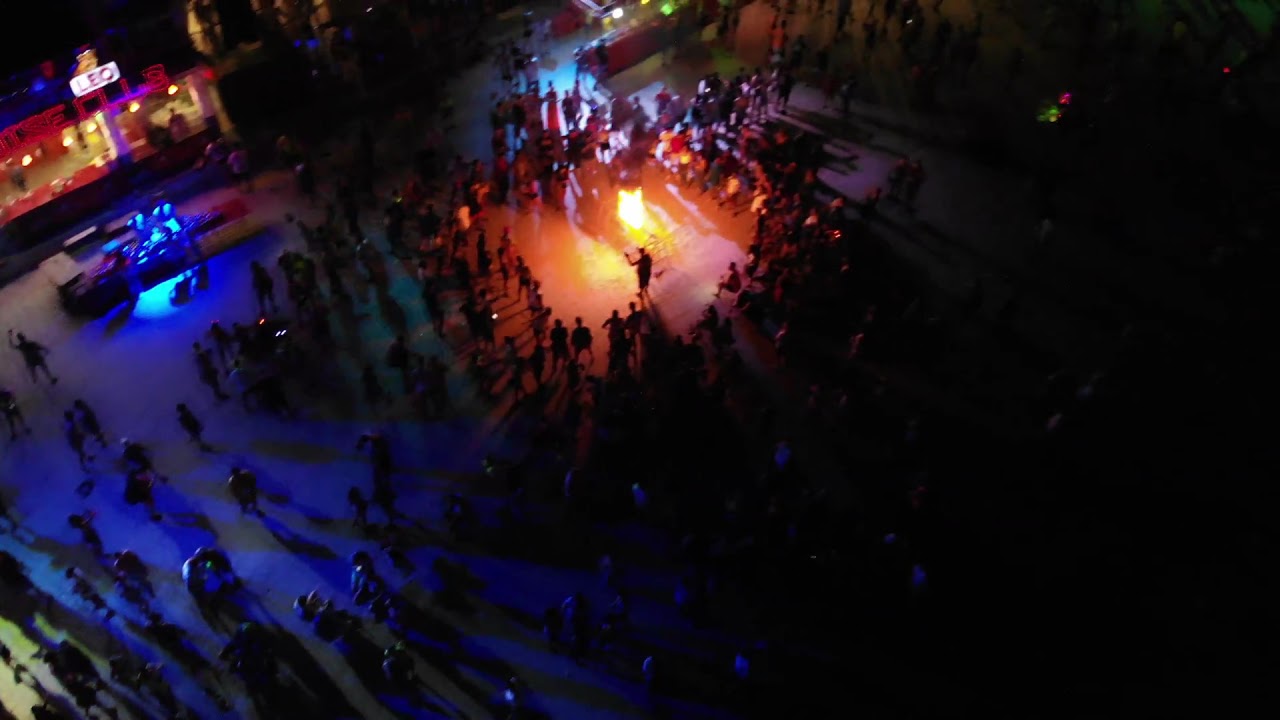This detailed, nighttime aerial photograph captures a dynamic public gathering. At the top center of the image, we see a crowd of people forming concentric circles around a dirt clearing, where a man stands with his arm raised, seemingly performing or speaking. Nearby, a bright light or fire source illuminates him. The crowd is dense at the center and gradually thins out toward the edges of the image, their colorful attire – in shades of white, blue, red, purple, pink, orange, yellow, black, and gray – adding vibrancy to the scene. To the left, a partially lit shopping plaza is visible, with a prominent building featuring a white, illuminated sign that reads "Leo." A vehicle, possibly a truck, is parked in front of this building. The photograph is taken from a drone, giving a comprehensive view of the event and emphasizing the realistic and representational style of the image. There is no text other than the sign, and the overall setting suggests a lively gathering in a public space.